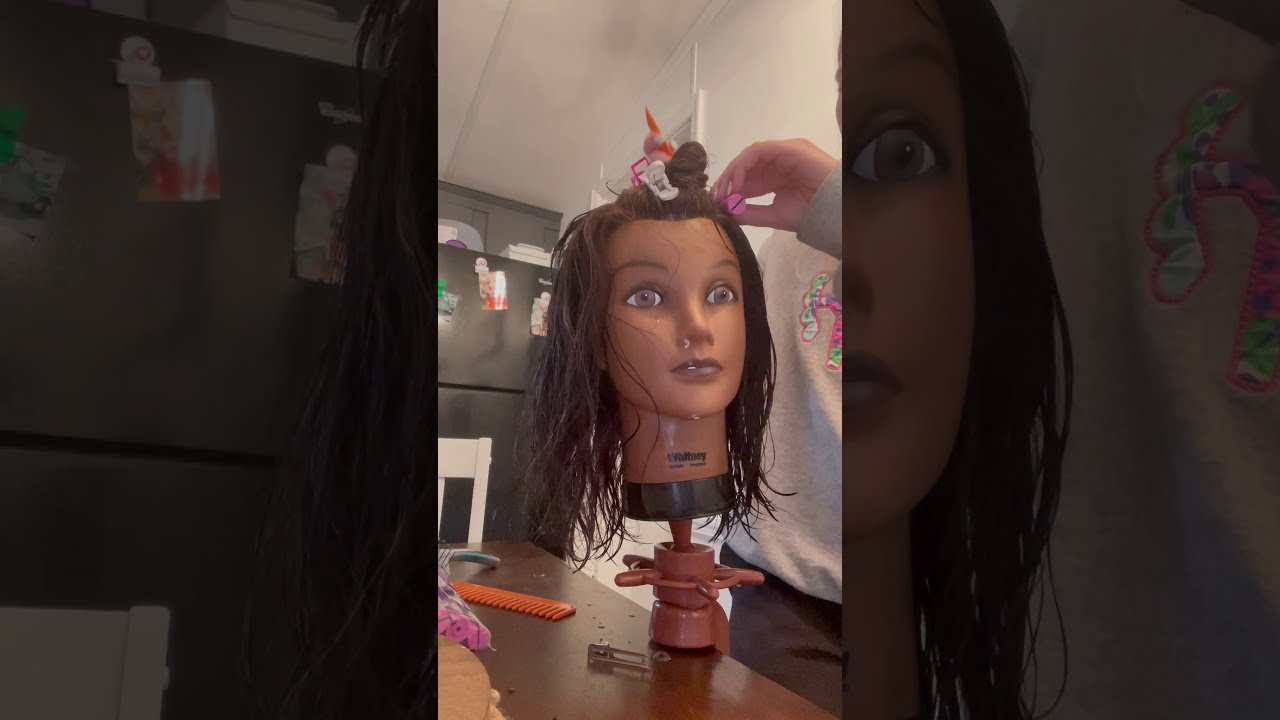The image is divided into three vertical sections, with the first and third sections showing darkened close-ups of the central picture. In the middle section, a room with white walls contains a brown table with a mannequin's head placed upon it. The mannequin, resembling an African American teenage girl, has light brown skin, big brown eyes, and brown hair parted on the side that falls below shoulder length. The hair is damp and partially styled, with a small knot on top and the sides hanging down. A Caucasian woman, dressed in a grey t-shirt and dark brown pants, is actively styling the mannequin's hair, inserting pink plastic curling rollers. Also on the table are an orange comb with large teeth, some clips, and various other items. At the end of the table, a white chair is visible, and in the background, there are black cupboards or possibly a refrigerator. The mannequin's base, a rotating brown stand, displays some unclear writing, likely indicating its manufacturer.